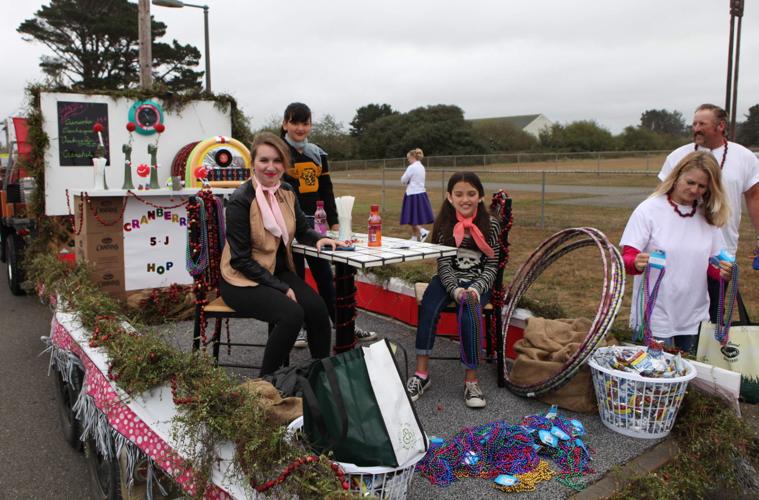The horizontal-rectangular image depicts a meticulously decorated parade float parked in a field. The float is a flatbed trailer hauled by a large truck. The flatbed is adorned with a gray carpet and festive decorations, including green grass garland with red beads and white banners trimmed in pink with white circles hanging above the tires. A large white table is set on the float, where an older woman with short, curled brown hair and a young girl with long brown hair are seated. They are dressed in classic 1950s attire, featuring leather jackets, scarves, full skirts, ponytails, and bright lipstick. Other people, similarly dressed in 1950s outfits, are scattered around the float, which is embellished with various retro items like hula hoops, pom-poms, and old-fashioned milkshake machines resembling a cafe setup. A jukebox and a vintage clock add to the nostalgic ambiance. A pile of purple and blue items and a sign that reads "Can Cranberry 5J Hop?" are positioned at the end of the truck. The scene evokes a lively and colorful mid-20th-century celebration.